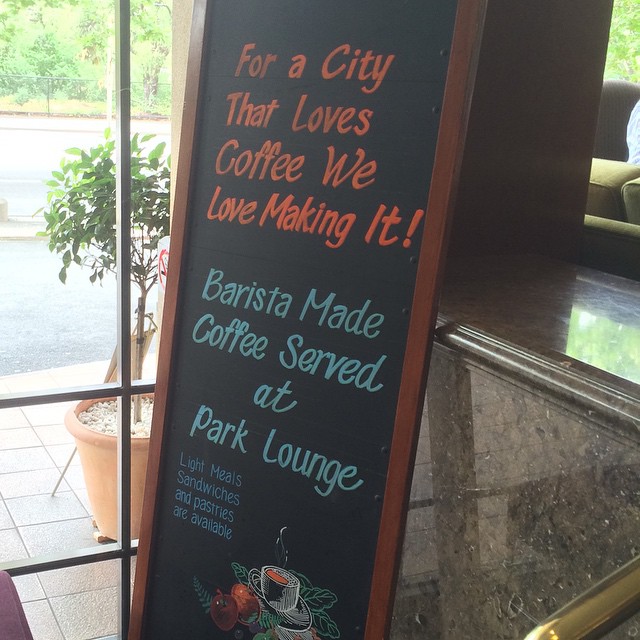This photograph captures a vibrant and detailed scene inside a cafe, featuring a prominent black chalkboard sign with a decorative frame. The chalkboard, which appears central in the composition, is filled with colorful text that reads from top to bottom: "For a city that loves coffee, we love making it." This phrase is written in a gradation of colors, starting with orange and transitioning to a turquoise-green hue. Beneath this, in blue lettering, it advertises "Barista made coffee served at Park Lounge," also mentioning the availability of light meals, sandwiches, and pastries. The bottom of the chalkboard is adorned with an artistic chalk drawing of a steaming coffee cup with a saucer, surrounded by apples and leaves to add a decorative touch. To the right of the sign is a dark granite or marble countertop, while to the left, a large window reveals a sidewalk outside with a potted tree. You can also glimpse a tiled sidewalk, a road or parking lot, and a fence line against a backdrop of green grass in the distance. The chalkboard leans against a half wall, part of which is mirrored, contributing to the intricate and inviting ambiance of the cafe.